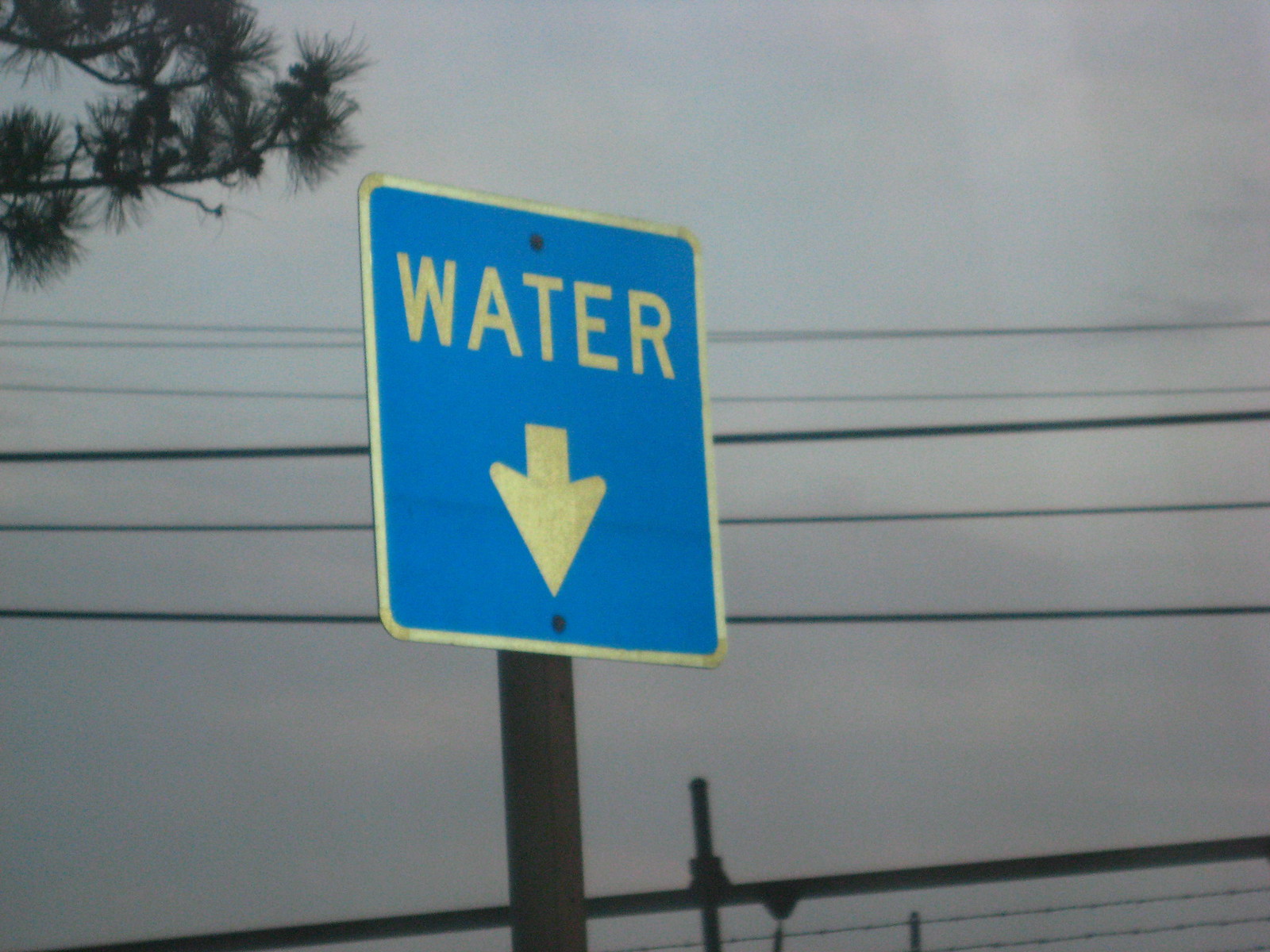The photograph captures a cloudy day with a light gray sky, interrupted by needle-like pine tree branches extending from the top corner, some adorned with pine cones. Dominating the scene are numerous utility elements; several telephone poles and intermingled power and internet lines crisscross the sky, amounting to a total of six distinctly visible wires. Centrally featured is a tall, brown wooden utility pole with a prominent blue square sign bordered by white trim. The sign reads "WATER" in white uppercase letters, with a matching white downward-pointing arrow beneath the text. Below and behind this pole, additional power lines and metal structures contribute to the dense web of infrastructure. At the bottom, a section of wired fencing adds further texture to the scene.